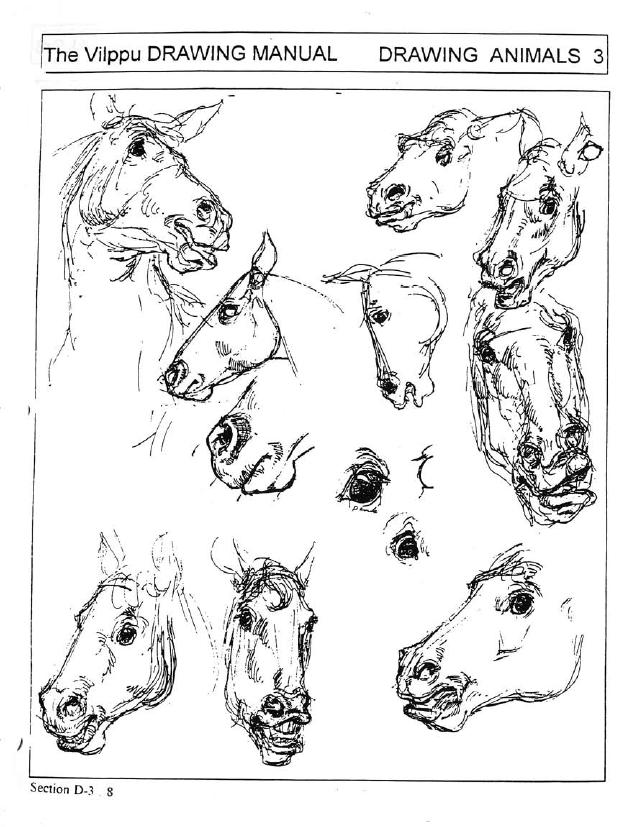This image depicts a page from "The Vilppu Drawing Manual, Drawing Animals Free," specifically section D-3, page 8. The page, set on a pure white background, showcases an array of roughly a dozen pen and ink sketches of horse heads enclosed within a black rectangle. These detailed illustrations capture various angles and expressions of horses, from full neck and head profiles to isolated features such as eyes and nostrils. The detailed nose sketches are prominently featured alongside several disembodied horse eyes near the center. At the bottom, each horse head is meticulously presented, including one looking left and another facing forward with an open mouth, depicting a range of perspectives and detailing to aid in understanding the anatomy and expression of horses.